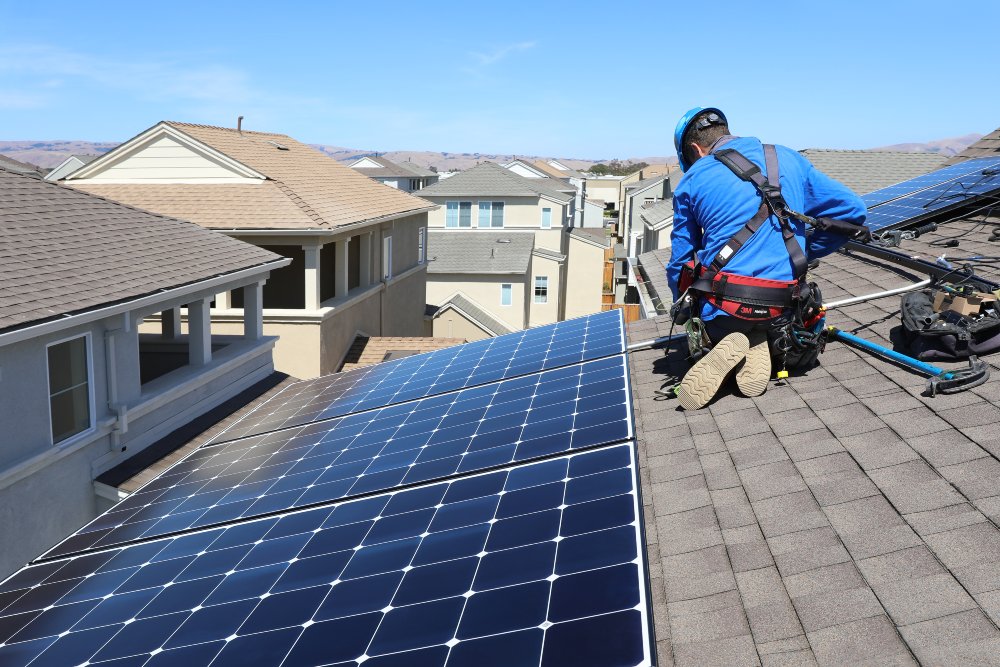In the image, a worker is installing solar panels on a densely packed residential rooftop. The worker, wearing a blue shirt, safety harness, and blue helmet with tan-soled boots, is positioned just above a row of solar panels that extends from the edge of the roof upwards. He appears to be working on a new row with conduit extending vertically from the existing panels before making a right-hand turn off into the background. His tool inventory includes a pipe bender and a basket of tools. Other homes with beige, tan, and gray shingles surround the scene, under a clear blue sky dotted with a few clouds. The man is visibly harnessed, as noted by a safety cable attached to his harness, ensuring his security while he works at height.